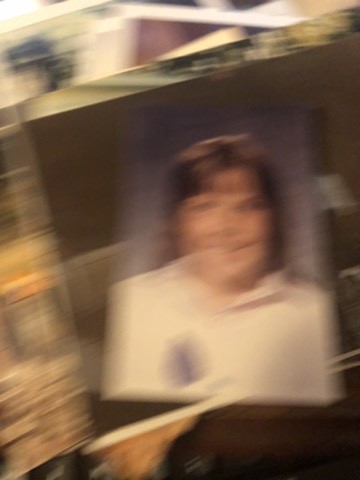A blurry, color photograph captures a stack of other photographs scattered across a surface. The top photo is a noticeably blurry class portrait featuring a person with dark hair and bangs. Despite the blur, the individual can be seen smiling. They are dressed in a white collared shirt adorned with a purple emblem or logo over the left chest area. The dimensions of this photo are taller than they are wide. Due to the significant blur, no text or additional details are legible, and there are no visible animals, plants, flowers, or trees in the image.